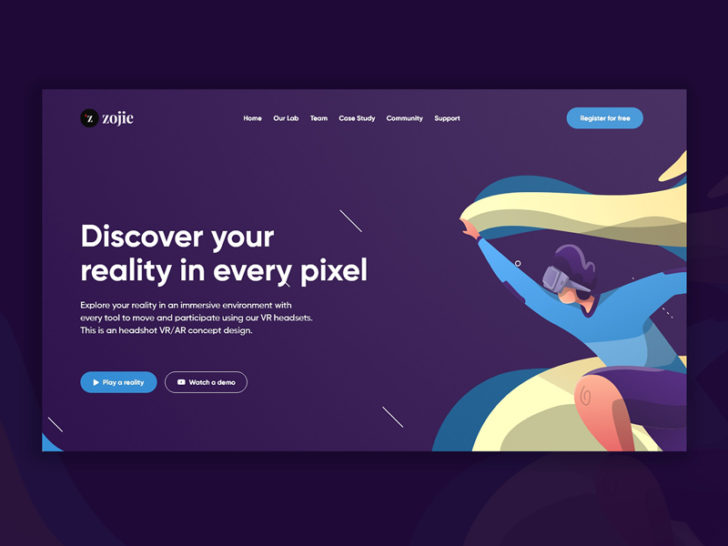**Caption:**

A detailed screenshot of a website from the company Zoji, characterized by a striking dark purple background and white text. The interface features a black outline of a computer screen, encapsulating the vibrant site. The top navigation bar lists categories such as Home, Our Team, Community Support, and Cross-Study, all in white text. In the upper right-hand corner, there is a prominent blue box prompting users to "Register," though the full details are partially obscured.

Central to the homepage is a bold white headline stating "Discover Your Reality in Every Pixel," accompanied by an explanatory subtitle: "Explore your reality in an immersive environment with every tool to move and participate using our VR headsets." This text introduces Zoji's VR/AR concept design.

Toward the bottom of the page, a blue, oval-shaped button labeled "Play a Reality" invites visitors to watch a demo, housed within a purple box. Additionally, an animated image of a cartoon character adds a playful element to the page. The character, sporting virtual reality goggles and appearing to run with a yellow flag, is dressed in purple pants and a blue top, perfectly coordinating with the website's color scheme.

Overall, Zoji's website efficiently combines vivid visuals and informative text to immerse users in their innovative VR/AR offerings.